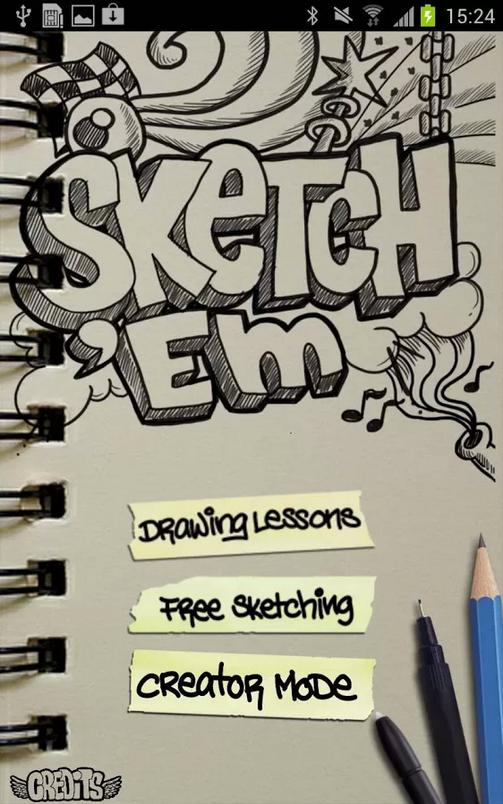This image features a vertical screenshot from an Android device displaying a spiral-bound sketchbook as the main background. The notebook, appearing as an off-white page, contains intricate sketches, including a checkered flag, a star-tipped magic wand, a pair of chains, a wave, and musical notes emanating from a horn. At the top of the sketchbook page, large bubble letters spell out "Sketchum" in two lines, with additional text detailing "Drawing Lessons," "Free Sketching," and "Creator Mode" taped onto the paper towards the bottom. In the lower left corner, the word "Credits" is displayed in white letters outlined in black, fashioned with wing-like symbols on either side. On the right side of the page, a light blue pencil and two black pens sit near the bottom. Across the top of the screen is the typical status bar icons found on mobile devices: a green battery symbol, a mute icon, and Wi-Fi strength indicator, with the time displayed as "1524". The background and drawing instruments are captured with the stylized elegance of a mobile screenshot.